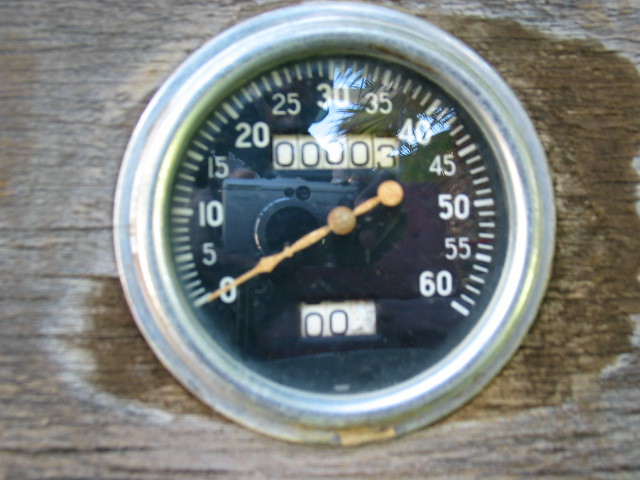This image features a prominently centered circular gauge, likely a speedometer, mounted on a weathered wooden surface with a distinguished gray patina. The gauge shows clearly defined increments of five, ranging from 0 up to 60, with intermediary tick marks for precision. At the center of the gauge, there is an odometer reading "3", accompanied by an additional meter below that reads "00" with a blank dial beside it. The bezel of the gauge appears to be aged aluminum, adding a vintage charm to the setup. The speedometer face is black with contrasting white numbers and markings, all protected under a glass lens. A notable aspect of the image is the reflection captured on the lens, revealing the photographer's silver camera with a prominent black lens and the faint silhouette of the person. Additionally, the reflection shows fan palms and telephone lines in the top right corner, adding a touch of the surrounding environment to the detailed composition.